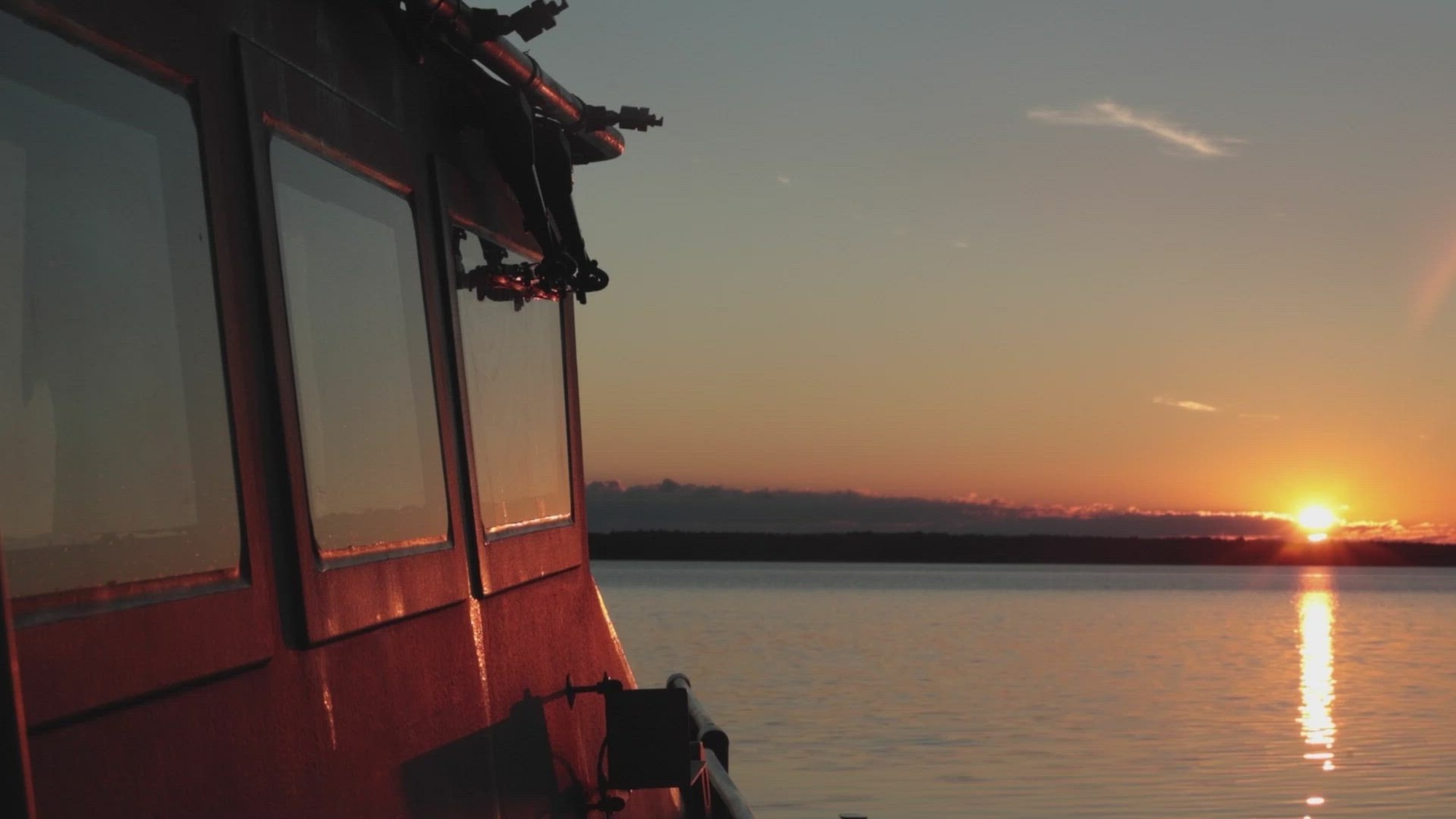This photograph captures a serene scene of a sunset over a vast, calm body of water, possibly a river or large lake. The setting sun, a brilliant yellow orb, illuminates the sky with a gradient of colors, transitioning from warm oranges near the horizon through lavender and into a darker blue towards the top. A small handrail and three square windows line the red-painted side of a well-maintained boat in the foreground on the left. The glassy water reflects the vibrant sky and the distant, dark landmass along the shore. Two thin, white clouds float near the sun, while a storm front seems to loom in the distant background, adding dramatic tension to the otherwise tranquil scene.